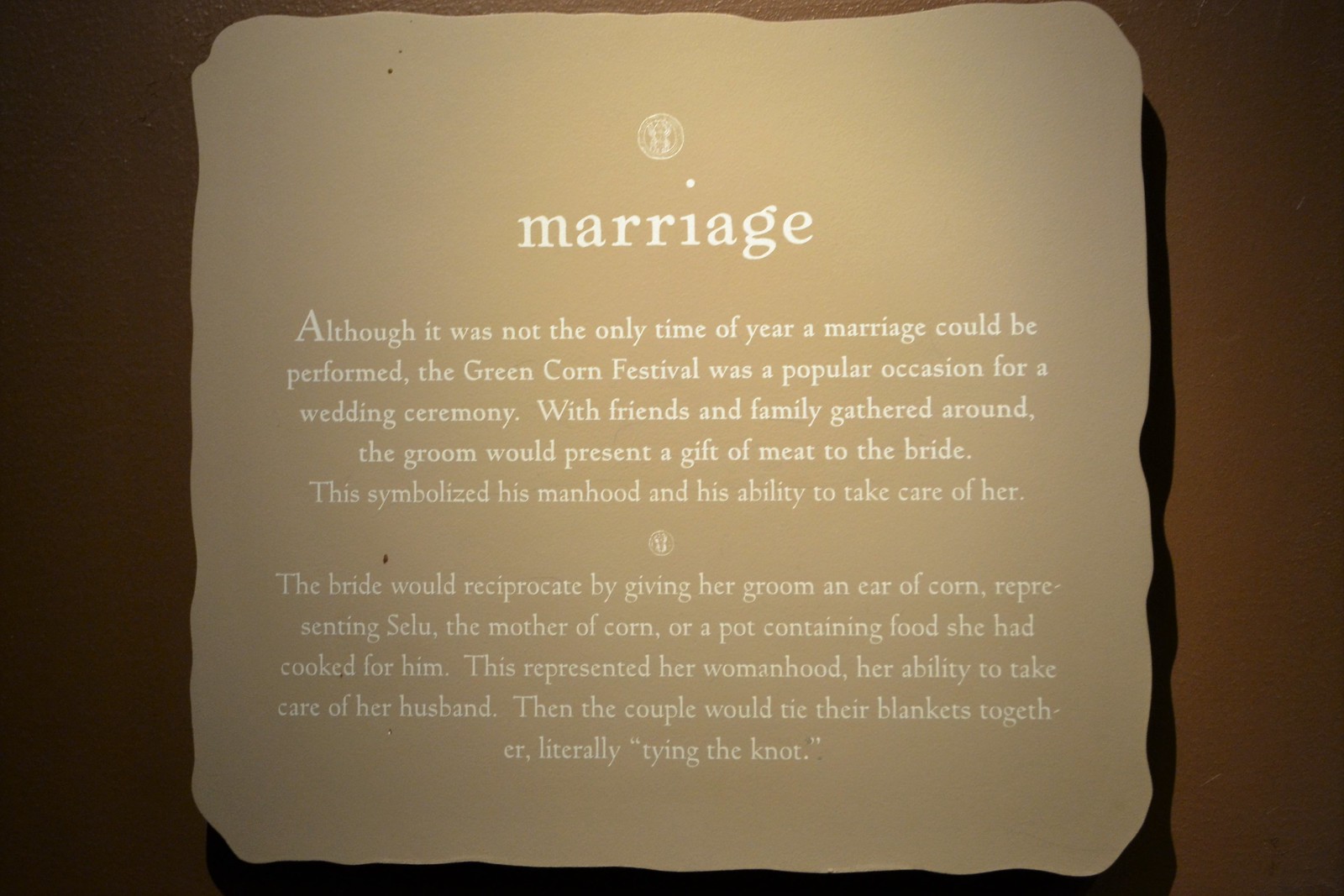This image is a photograph of a horizontally rectangular plaque with a light tan background and curvy edges, mounted on a dark brown wall. At the center top, there is a circular white stamp above the title "marriage" written in lowercase white letters. Below the title, in two centered paragraphs, the text explains that although marriage could be performed at any time of year, the Green Corn Festival was a popular occasion for wedding ceremonies. During this event, the groom would present a gift of meat to the bride, symbolizing his manhood and ability to provide for her. In return, the bride would give the groom an ear of corn, representing Silu, the mother of corn, or a pot of food she had cooked, signifying her womanhood and capability to care for her husband. The ceremony would culminate with the couple tying their blankets together, symbolically "tying the knot." Another circular stamp is located between the two paragraphs of text.